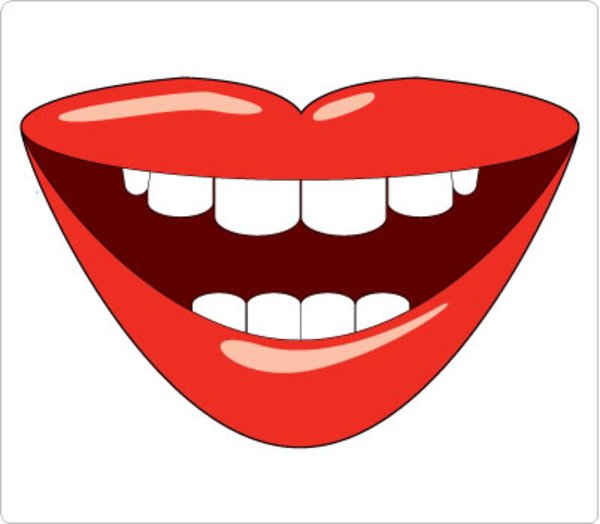This image is a detailed color illustration of a woman's slightly open and smiling mouth. The lips, prominently outlined in a vivid red, exude a shiny appearance, highlighted by off-white accents on the upper left and lower center portions. The smile reveals white teeth—six on the top row and four on the bottom—against a dark burgundy inside. The background is entirely white, giving a striking contrast to the bright red lips. Surrounding the entire image is a thin, gray hairline border with rounded corners, lending it a clean, framed appearance. The artwork, reminiscent of pop art or modern graphic design, exudes a cheerful and friendly expression.